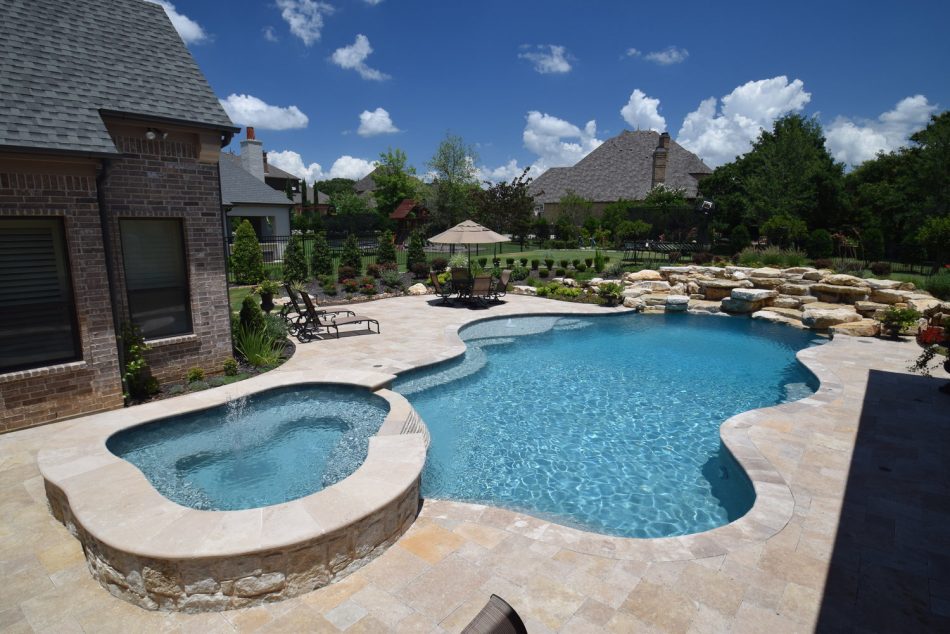The image showcases a stunning backyard scene featuring an unconventional, cloud-shaped in-ground pool with wavy, curved edges and a deep blue hue. Adjacent to the pool on the left is a slightly elevated jacuzzi adorned with a beautifully crafted stonework wall around its rim. Both the pool and jacuzzi are enclosed by a sleek black metal fence. At the far end of the pool, a man-made rock formation serves as a captivating waterfall installation, adding to the tranquil ambiance. The backyard is part of a sizable, well-landscaped property in front of a grayish-red brick mansion with a dark gray roof. Several other similarly designed buildings are visible in the background. Complementing the scene are meticulously manicured bushes, green trees, and a blue sky with fluffy white clouds. The recreational area is equipped with deck chairs, a table with four chairs around it, and an umbrella, perfect for outdoor relaxation. The entire setup suggests a professionally designed landscape, emblematic of a luxurious residential area.